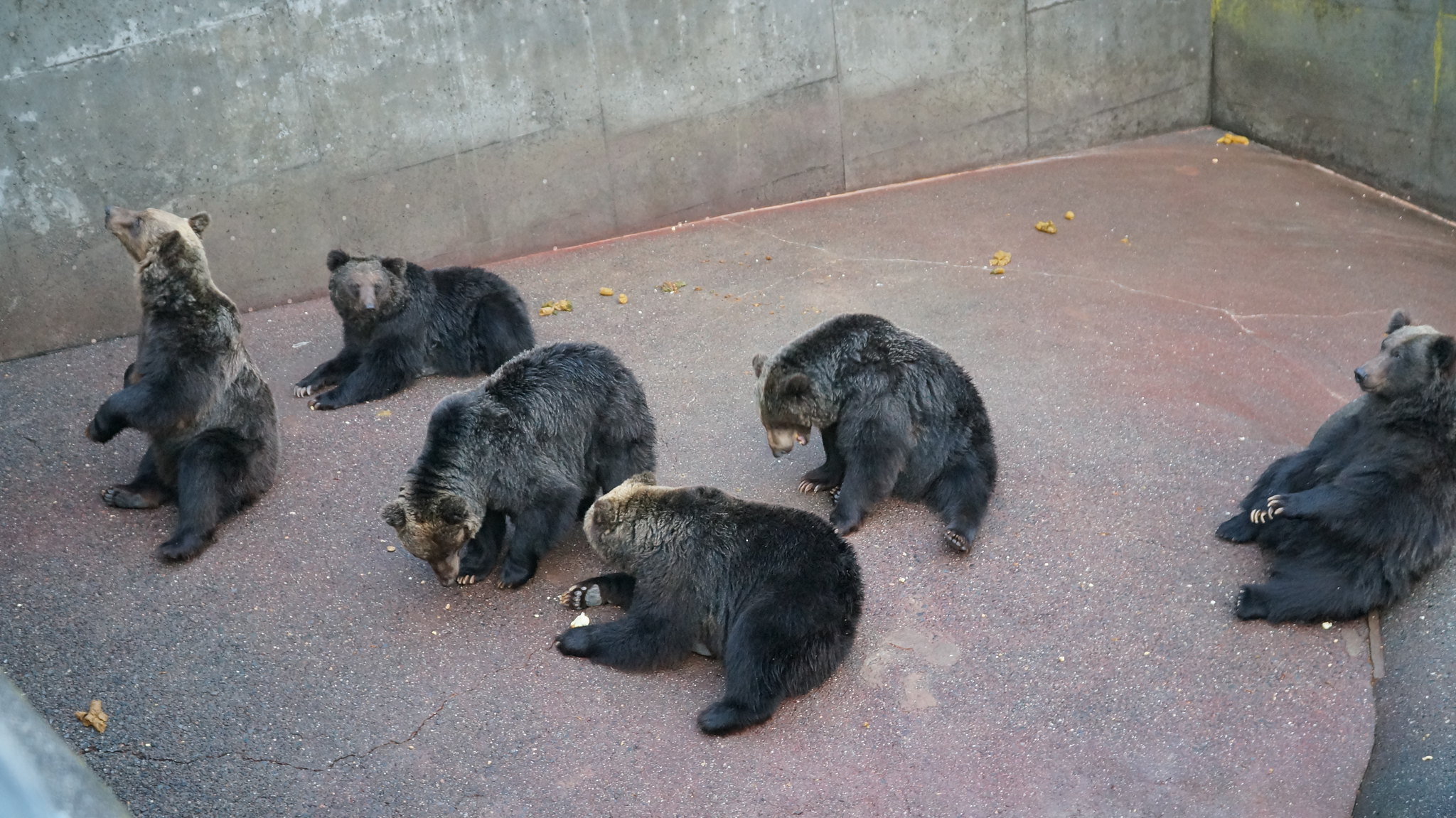This image features six black bears in captivity within an enclosure that appears to be part of a zoo. The enclosure has high concrete walls, sloped asphalt pavement, and a cracked concrete floor. The environment looks grim and unwelcoming, with no visible trees or water for the bears. Scattered bits of yellowish-brown material cover the ground. 

The bears are mostly seated or lying down. One bear, distinguishable by a tan stripe on its head, is sitting with its back against a rock support, looking upwards. Another bear also has tan fur on its head and is looking up. Three bears are focused on eating something off the ground, and one bear is simply lounging. All the bears share dark fur with lighter brown fur around their muzzles and foreheads, and they all have light-colored claws. The overall setting looks dirty and confined, hinting at an uncomfortable living situation for the bears.